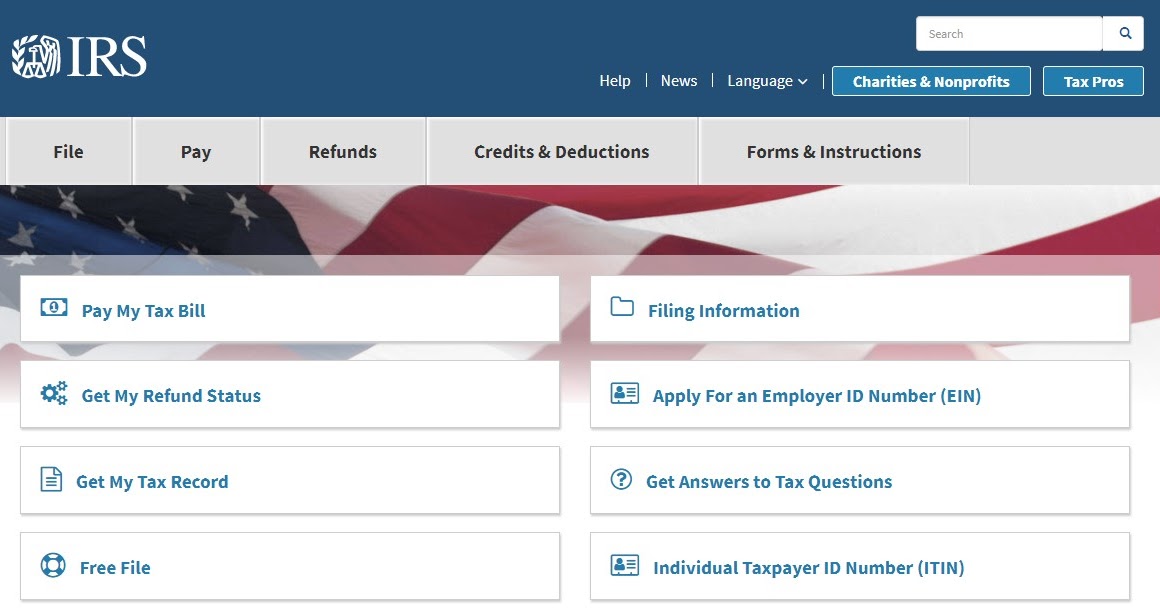This image is a detailed screenshot of the IRS's official website. At the top left corner, the page prominently features the IRS emblem alongside the letters "IRS". To the right, there is a navigation banner with tabs for "Help," "News," and "Language Options." Alongside these tabs, there are two additional buttons labeled "Charities and Non-Profits" and "Tax Pros," accompanied by a search bar and a search button at the very top for user convenience.

Beneath this navigation banner, another set of options is displayed, offering links to various sections of the site such as "File," "Pay," "Refunds," "Credits and Deductions," and "Forms and Instructions."

Dominating the central part of the page is an image of an American flag, subtly used as a background for eight user options. The design is clean and functional, with white boxes featuring blue text, superimposed on a semi-transparent background to ensure readability.

The eight options are strategically placed in two columns. In the first column from top to bottom, the options are: 
1. "Pay My Tax Bill"
2. "Get My Refund Status"
3. "Get My Tax Record"
4. "Free File"

In the second column from top to bottom, the options are: 
1. "Filing Information"
2. "Apply for an Employer ID Number (EIN)"
3. "Get Answers to Tax Questions"
4. "Individual Taxpayer ID Number (ITIN)"

Overall, the design is user-friendly, featuring a mix of intuitive navigation and visually appealing elements, typical of a well-structured government website.